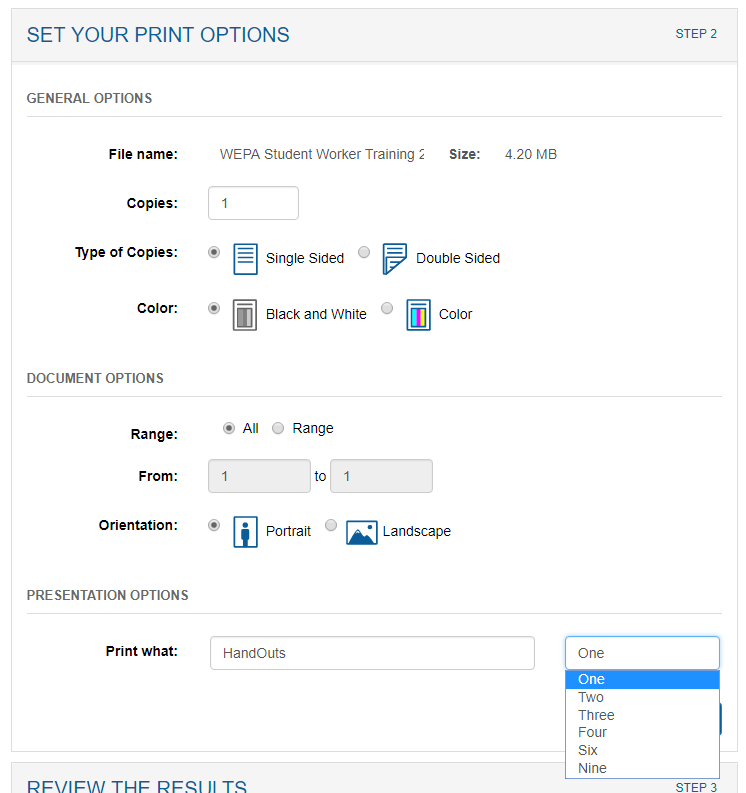Screenshot showing the "Set Your Print Options" webpage interface.
 
At the top of the screen, within a grey rectangular header, it reads "Set Your Print Options." On the right side of this same grey header, "Step 2" is displayed. Beneath this, the background of the webpage changes to white and remains so until the very bottom where a grey strip is visible. On the left side of this strip, it states "Review the Results," while "Step 3" is shown on the right.

Dominating the central white background is a series of print settings. The section titled "General Options" allows users to enter details such as the file name, the desired size, the number of copies, and the type of print (e.g., single-sided or double-sided, black and white or color). The current selections indicate single-sided printing, one copy, in black and white.

A faint grey line delineates the next segment, labeled "Document Options." Here, the option "All" is visible, followed by a field that specifies printing from page 1 to page 1. Further down, under "Orientation," users can choose between "Portrait" and "Landscape," with the current selection being "Portrait." At the bottom section, there is an option titled "Print What."